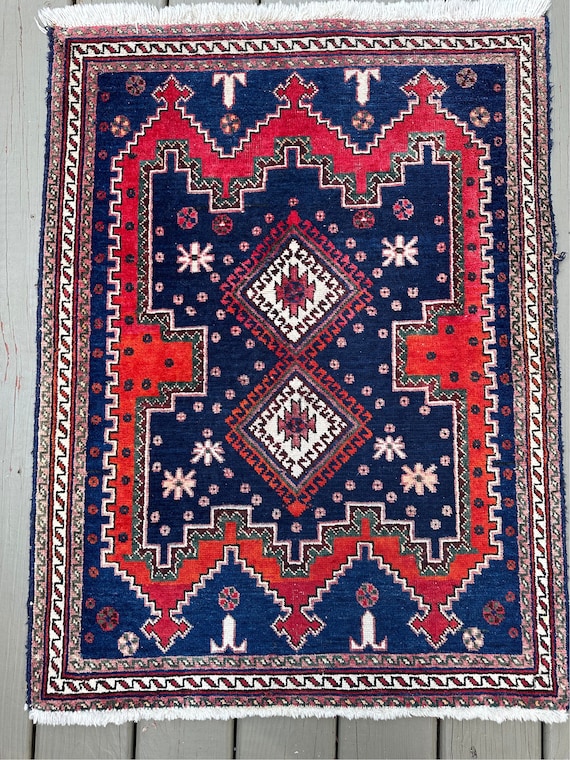This image captures a detailed and ornate area rug placed atop gray-washed wooden planks, which could be part of a deck. The rug predominantly features a rich palette of reds, blues, whites, and burgundy colors. Intricate patterns adorn the rug, including diamond shapes in the center and a motif that suggests tall peaks or castle-like structures around the edges. The fringe on either end of the rug is white, though one side appears to be unraveling, hinting at its frequent use and age. Some elements of the design evoke imagery that could be reminiscent of a family crest, and there are intricate circles, flowers, and letter T shapes interwoven throughout. Overall, while the origins of the rug could be speculated to be from either the Southwest or regions like India or Pakistan, its vivid detailing and focal presence in the image make it a strikingly beautiful piece.